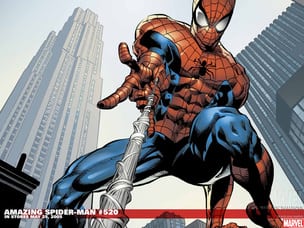The image is a comic book-style illustration of Spider-Man viewed from below, giving the impression that he's slightly above and looking down at the viewer. Spider-Man is depicted in a very muscular form, showcasing detailed six-pack abs and defined leg muscles. He wears his iconic costume, consisting of red and blue sections with a black spider emblem on his chest. His red mask features the characteristic spider eyes.

Spider-Man's body posture suggests that he has either just finished a jump or is about to leap again, with his legs bent and arms extended forward. From his wrist, he is shooting webbing aimed toward the viewer, extending off the screen.

In the background, the Empire State Building towers prominently behind Spider-Man, reaching up into the sky, and another tall skyscraper is visible to his right. Additional buildings can be seen further in the background, contributing to the urban setting.

At the bottom left of the image, a red banner with white text reads "Amazing Spider-Man number 520," and there is a red rectangle with white text in the lower right corner, bearing the Marvel logo. Some smaller text is present below the banner, but it is too small to be legible.